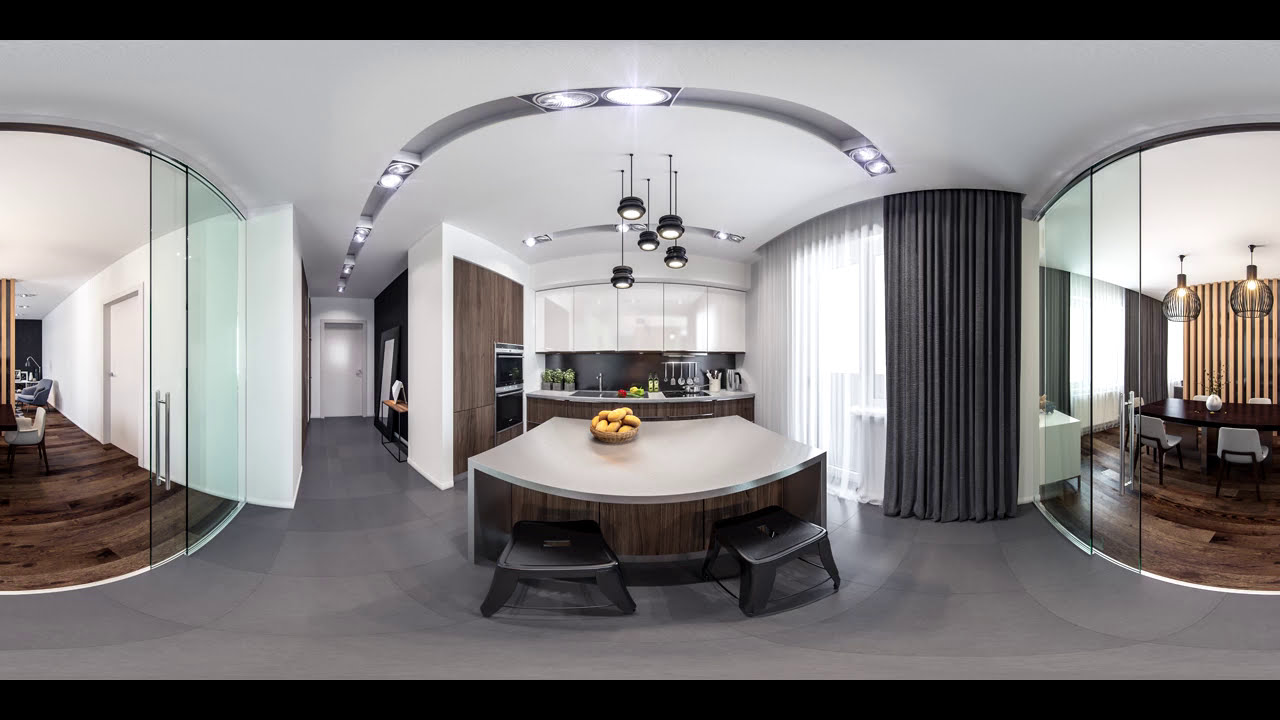This 360-degree panoramic image reveals the interior of a high-end, modern kitchen and dining room area in a sleek condo or apartment. The kitchen, directly in front of us, features a light gray breakfast bar with two gray stools and hanging modern lights above. The bar top holds a bowl containing fruit or possibly bread. The floor is a solid medium gray with alternating light gray and medium gray rectangles. Glossy white cabinets line the walls, accompanied by a wood-paneled, inset refrigerator that matches the wood accents around the oven range.

The kitchen sink area boasts large hanging utensils and black accents. A prominent feature is the set of sheer white curtains that let in light, paired with dark gray curtains for blocking light. A black, modern chandelier hangs from the ceiling, adding a touch of sophistication.

On either side, the dining room is visible, accessible through sliding glass doors. It features a dark hardwood floor, a black table, and contemporary white chairs. Tall, floor-to-ceiling windows are adorned with matching curtains from the kitchen area. Additional lighting in the dining room includes fancy sconces, enhancing the refined and luxurious ambiance of the space. The room appears exquisitely clean, with the overall design exuding an expensive and meticulously crafted feel.